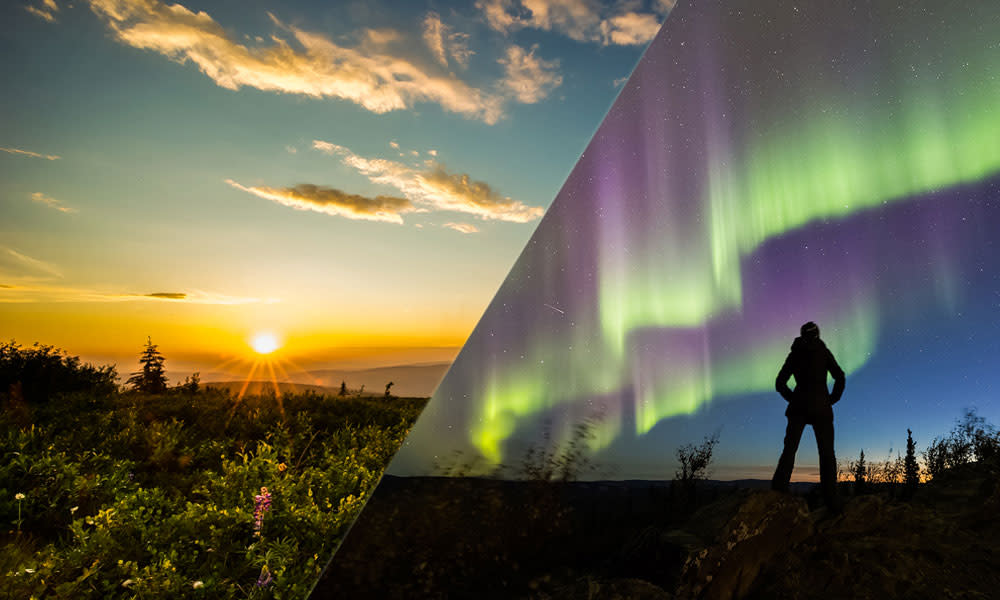The image is a split photograph divided diagonally, depicting two contrasting times of day. On the left side, it shows a breathtaking sunrise with a bright orange sun emerging over a slight mountain or hill range. The sky is a clear blue with scattered white, puffy clouds, and the landscape below features a forest area with various sizes of trees, a grassy field dotted with pink and yellow flowers, and some small shrubs. This side is bathed in the golden hues of early morning light.

On the right side of the image, it captures a nighttime scene illuminated by the Northern Lights, showcasing vibrant purples, greens, and blues dancing across the sky. In the foreground, silhouetted against the aurora, stands a figure, potentially a slim woman with long hair, wearing pants and a shirt, with her hands on her hips. The ground beneath her is shadowed, dotted with small shrubs, and the overall atmosphere evokes the quiet majesty of the night.

The juxtaposition of the two scenes suggests the same location at different times, emphasizing the beauty and grandeur of nature from dawn to dusk.